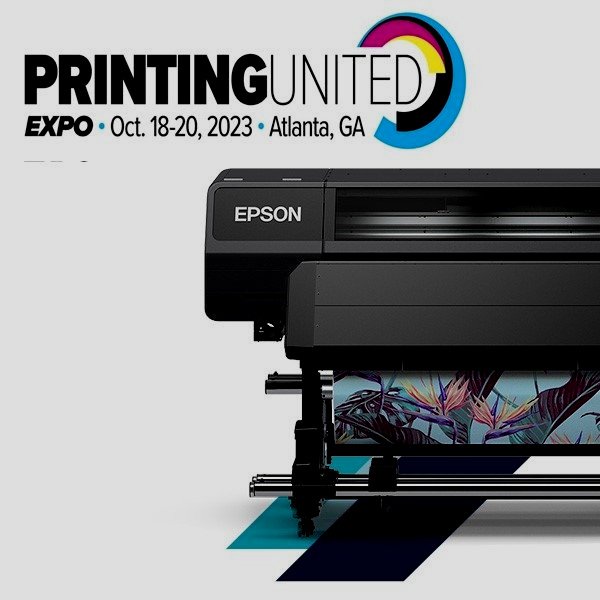This is an advertisement for the Printing United Expo on a grey background. At the top, the ad features the "Printing United" name and logo, the latter consisting of a blue three-quarter circle with black, yellow, and pink segments inside it. The text prominently announces the event dates, October 18th through 20th, 2023, in Atlanta, Georgia.

Dominating the middle of the advertisement is a large, black, rectangular Epson printer. The printer has a smaller rectangular feeding tray at the front and displays the white "Epson" logo. A vibrant, tropical print featuring a blue background and colorful tropical flowers is emerging from the bottom of the printer. Below the printer, silver bars stretch across, positioned just above the wheels. The overall background includes a dark cream color blending into different sections of the image, providing a subtle contrast to the prominent elements of the advertisement.